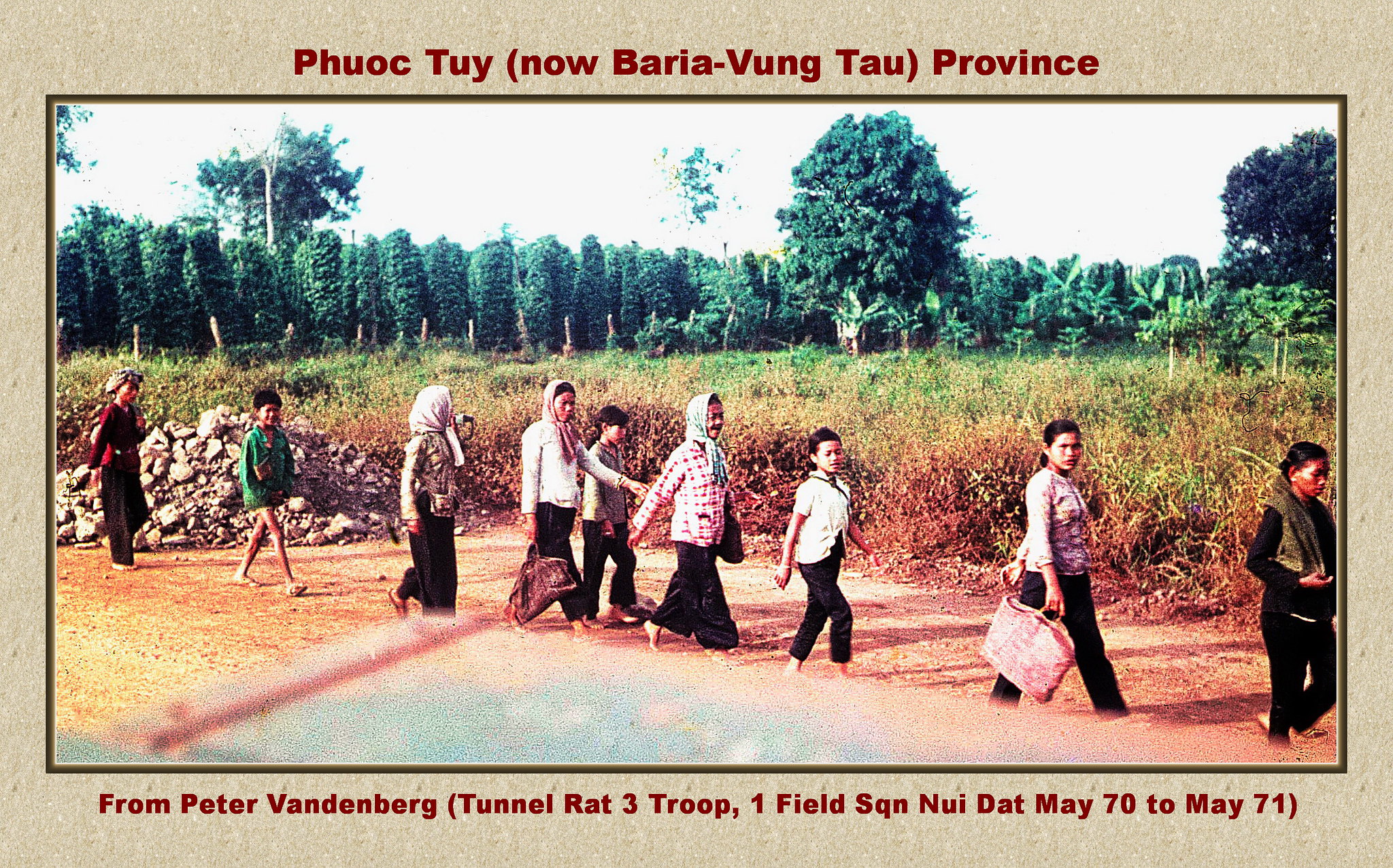This image, a rectangular photograph from the 1970s, depicts a line of 10 Vietnamese women and children walking down a dirt road surrounded by trees and grass, suggesting a rural setting during the Vietnam War. The caption at the top reads "Phuoc Tuy, now Baria Vung Tau Province," and at the bottom, "From Peter Vandenberg, Tunnel Rat 3 Troop, 1 Field Squadron, Nui Dat, May 70 to May 71." The individuals, some carrying bags, are primarily dressed in black pants or skirts, with a mix of head wraps and pulled-back hair. The mood appears peaceful rather than distressed, as they look either at the camera or ahead. The photograph was possibly taken from a truck.